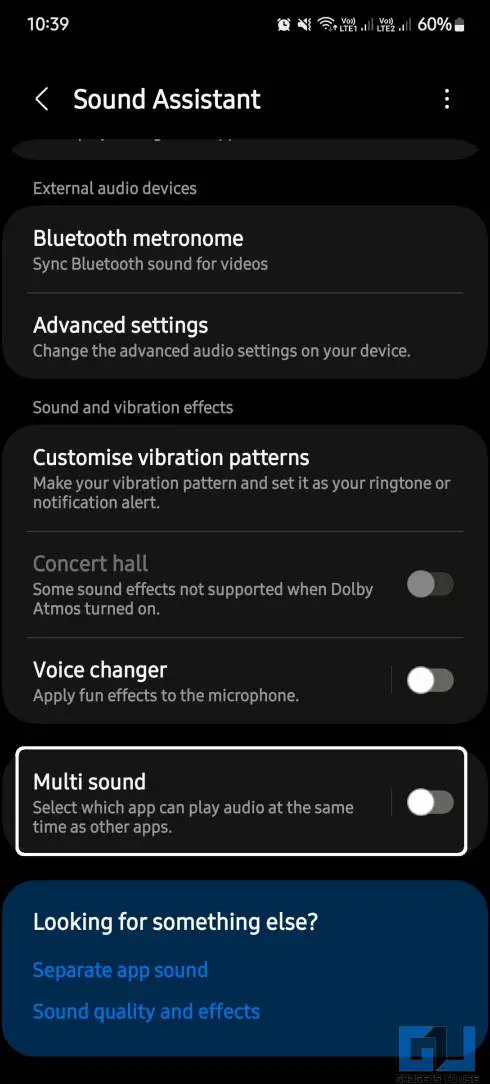The image is a screenshot of a mobile phone displaying the "Sound Assistant" section. The mobile phone features a black background, including a black status bar at the top. Located in the top left corner of the status bar is the time, set at 10:39. On the top right, multiple icons are visible, including a battery icon showing a 60% charge.

The "Sound Assistant" page contains the following rows and features:

1. **Bluetooth Metronome** - This is the first row.
2. **Advanced Settings** - Positioned in the second row.
3. **Customized Vibration Patterns** - Occupying the third row.
4. **Concert Hall** - Found in the fourth row; this option is not toggled on.
5. **Video Changer** - The fifth option, which is toggled on.
6. **Multisound** - The sixth row, which is toggled off and encased in a white box.

Below the "Multisound" row, there is a navy blue tag with the title "Looking for something else" in white text. Following this, there are two lines in blue text that read "Separate app sound" and "Sound quality and effects."

In the bottom right corner of the screen, there appears to be a watermark, seemingly the letters "GU."

This descriptive caption intricately outlines the visual and textual elements present in the screenshot, providing a thorough understanding of its contents.